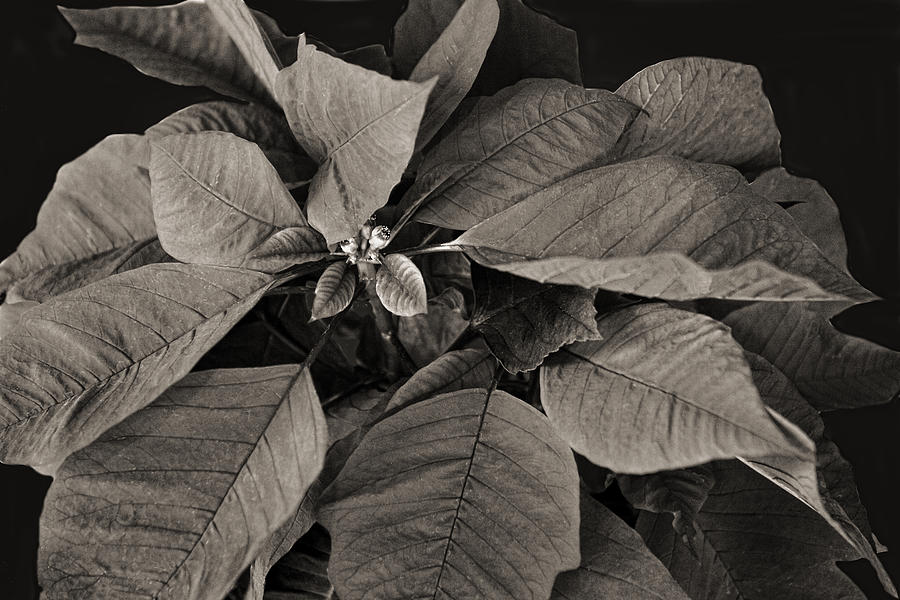The black-and-white photograph captures a detailed botanical study of a single plant, possibly resembling a poinsettia due to its distinctive leaf shape. The plant features large, wide, and crumply leaves that appear gray in the grayscale image. These leaves grow in clusters around a central stem, displaying a symmetrical pattern with prominent middle veins and diagonal horizontal veins. In the center, smaller leaves and two tiny, whitish buds can be seen, indicating the early stages of flowering. The background is completely black, providing a stark contrast that highlights the intricate details and textures of the plant's papery leaves spreading out in a circular fashion.